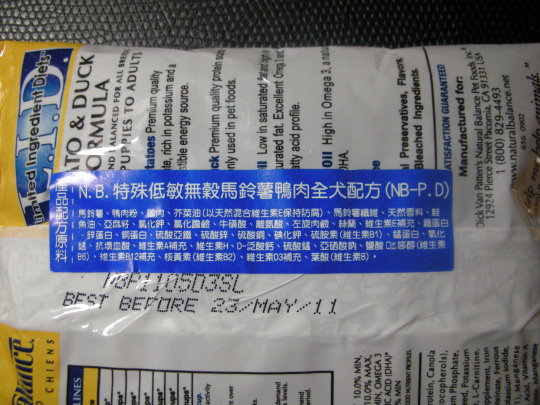This is a detailed photograph of a food package resting on a black surface. The primary color of the package is white, adorned with black text and accented with yellow squares. A prominent blue sticker runs down the center of the package, featuring white characters. A partial nutrition label is visible, showing black font, and the package is stamped with a "Best Before 23rd May 11" date. Notably, the text "Limited Ingredient Diet" and "Duck Formula" are displayed, indicating a specialty pet food. Additional black text at the bottom mentions it is "manufactured for Dick Van Patten's Natural Balance Pet Food Inc." The image also reveals phrases such as "Premium Quality Protein Used in Pet Food," "Rich in Potassium," and "Suitable Energy Source." The letters "NB" and other text appear, some in Chinese, suggesting an internationally distributed product. The overall impression is that this is a package of high-quality dog food designed for specific dietary needs.